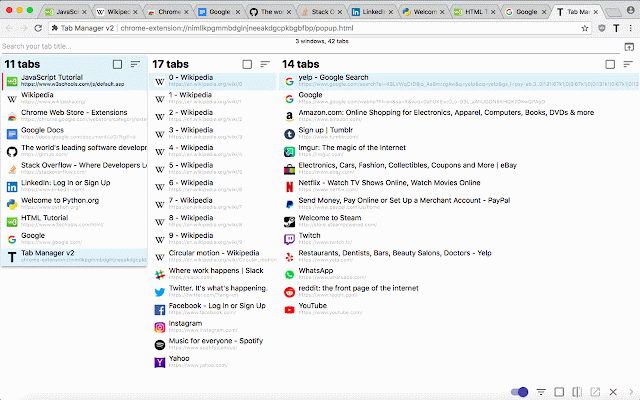A detailed screenshot of a desktop or laptop screen displaying the Chrome browser with a light gray top bar and a white background. Multiple tabs are visibly open: Wikipedia, Chrome Web Store, a Google Doc, Stack Exchange, LinkedIn, an HTML page, Google Search, and one titled Tab Manager. The active tab, Tab Manager, is emphasized, showing its URL as 'chrome-extension://...'. Below the URL bar are three columns. The first column, labeled "11 tabs," lists all the mentioned open tabs. The middle column, labeled "17 tabs," predominantly contains Wikipedia tabs, with nine or ten entries. The third column, labeled "14 tabs," includes various entries such as Google searches, Imgur, and Netflix.